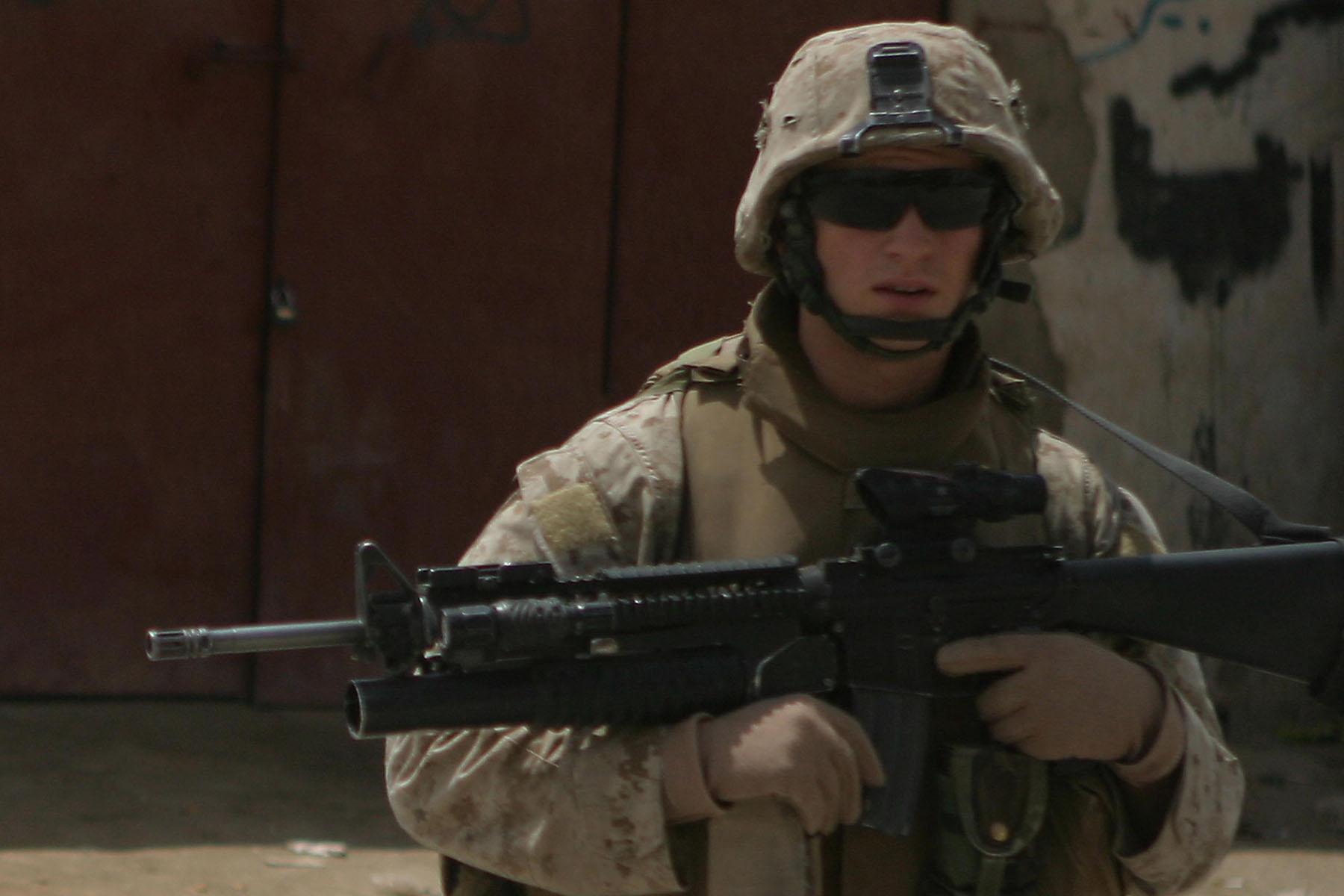The color photograph features a soldier clad in desert camouflage, dominated by light tans and browns, evocative of desert military operations. The soldier stands prominently in the center, gripping a large, black and silver machine gun with both hands. The gun, equipped with a short scope, is oriented to the left, its strap looped securely around his neck. He wears tan gloves that cover his hands completely. His face is partially obscured by very dark sunglasses, rendering his eyes invisible, and a black chin strap secures his helmet in place. An attachment piece for equipment, possibly for night-vision, sits atop his helmet. His intense gaze is directed straight at the camera.

In the background to the left, a large wooden structure—possibly a door or wall—crafted from dark, almost reddish wood, stands out. The overall setting, apparently sunny due to the washed-out colors, suggests an outdoor location. The image elicits a sense of purpose and readiness, characteristic of a military professional in a deployed environment.